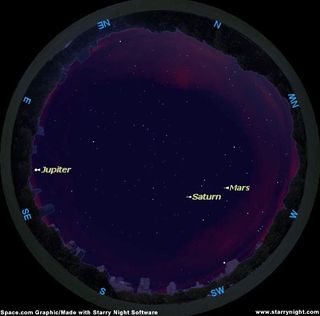The image is a detailed digital illustration simulating a view through a telescope aimed at outer space regions. The illustration is set against a black square background, framing a circular view bordered by a dark gray rim. Around this circular frame, light blue letters indicate directional positions: N for North, NE for Northeast, E for East, SE for Southeast, S for South, SW for Southwest, W for West, and NW for Northwest. 

Within the circle, the central area is depicted with rich dark purple hues, transitioning to lighter shades of pink and lavender, suggesting the presence of cosmic gases. Scattered throughout are small, white, dotted stars, enhancing the celestial atmosphere. Three planets are labeled inside the circle: Jupiter, Saturn, and Mars, each name written in white to stand out against the darker background.

Additionally, the image includes annotations in the lower right and left-hand corners, mentioning that it is a "Space.com graphic made with Starry Night software" and providing the website www.starrynight.com for further reference.